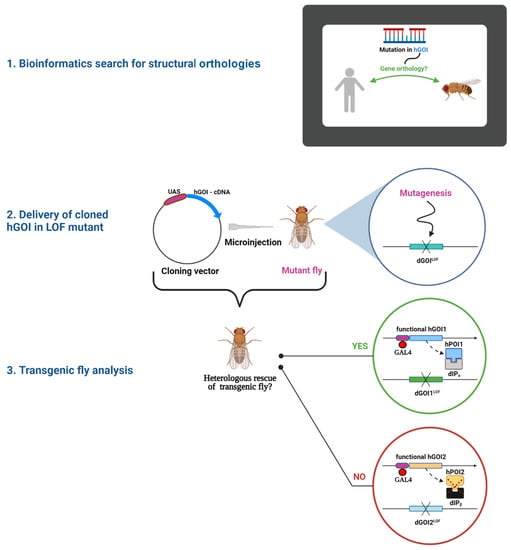The image is a detailed diagram with a white background, surrounded by a black striped outline. At the center, a series of bars topped with red lines and connected to a base represented by a dark green line are depicted. Behind these bars, there is partially visible text that might read "Mutation in H 601," though it is hard to read. A green arrow with points at both ends separates a gray silhouette of a man on the left from a bumblebee on the right.

To the left side of the image, there are three lines of text labeled one, two, and three. The first line reads "Bioinformatics search for structural orthologies." The second line, while not always consistently described, seems to involve the cloning or mutation of a gene. The third line mentions "Transgenic fly analysis."

Four large circles with text and imagery are positioned centrally. The details in these circles include descriptions such as "mutagenics," "functional CX2," and "microinjection," along with related graphics, though the specifics are hard to distinguish. Near these circles, there are additional images of insects, specifically flies, with some undergoing an injection, labeled "cloning vector and mutant fly" and "heterologous rescue of transgenic fly."

On the right part of the image, blue, green, and red color coding might indicate different stages or components of the process depicted in the diagram.